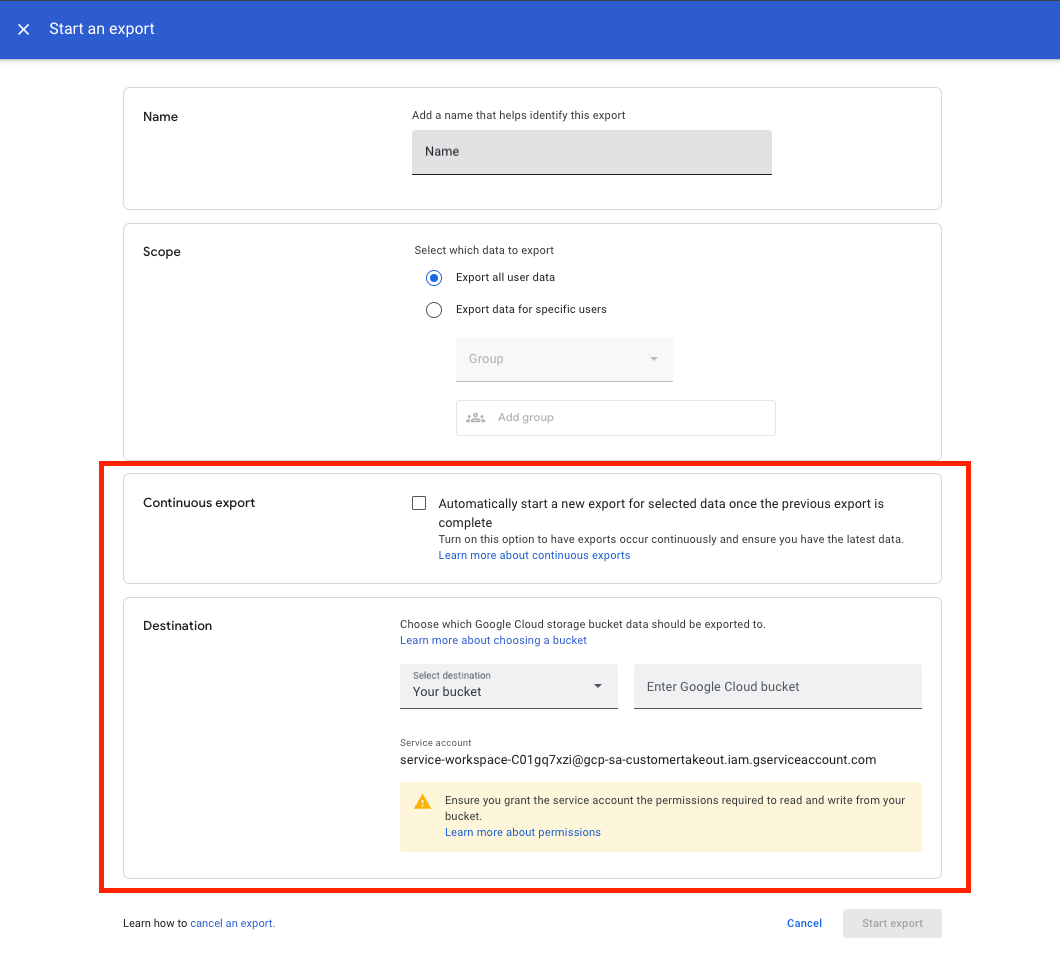This image appears to be a screenshot from a web interface for exporting user data. The top section of the image features a dark blue header with a thin black line along the very top. In the top left corner of this header, a white 'X' is visible next to the white text that reads "Start an export."

Below the header, the background is entirely white. Directly beneath the letter 'P' of "export" in the header, there is a long rectangular field. This field has the label "Name" in the left corner and the prompt "Add a name that helps identify this export" in the center. Inside this field, there is a light gray box with the word "Name" written in black text.

Further down, there is a space followed by another larger rectangular field labeled "Scope" in the left corner. In the center of this field, it says "Select which data to export." This section includes two radio button options: the first is a circle with a black outline, white interior, and a blue center labeled "Export all user data." The second option is a white circle with a black border labeled "Export data for specific users."

Below this section, there is a gray bar labeled "Group" which has a dropdown tab. Beneath this bar, a white rectangular box is labeled "Add group."

The remaining part of the page is occupied by a larger section outlined in a thick black border, almost as if it has been highlighted or circled. Within this area, a smaller rectangle contains the text "Continuous export" on the right, accompanied by explanatory information about this feature. Moving down, the next segment is labeled "Destination" on the left with two lines of relevant information.

This section continues with two more gray dropdown tabs. Below that, there is a "Service account" section displaying an account number, followed by a tab for "Permissions."